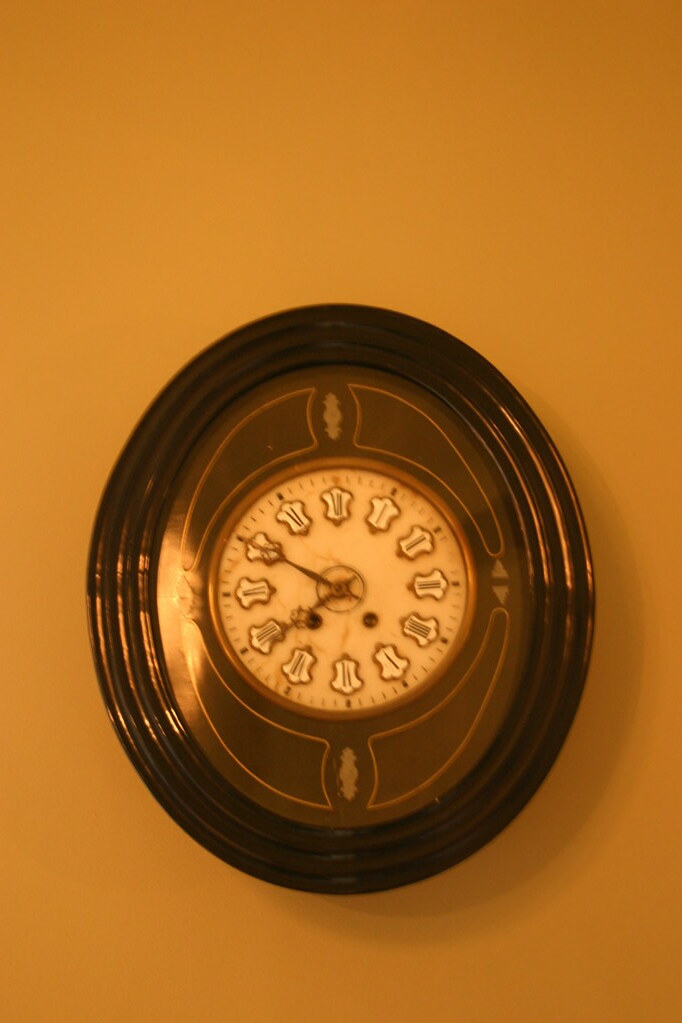The image showcases a detailed photograph of an oval-shaped wall clock hanging on a mustard-colored wall, emitting an orange hue. The clock features a prominent dark brown, three-lobed wooden frame. Encircled by this frame is an ivory clock face embellished with intricate gold filigree and highlighted by brown Roman numerals that stand out on small ivory bell-shaped cutouts, subtly distinguished by a lighter hue. The clock hands, ornate and decorative in design, indicate a time of approximately 3:50 with the shorter hand near the VIII and the longer hand pointing at X. The overall appearance of the clock evokes a sense of vintage charm, enhanced by the warm, reflective lighting of the room.